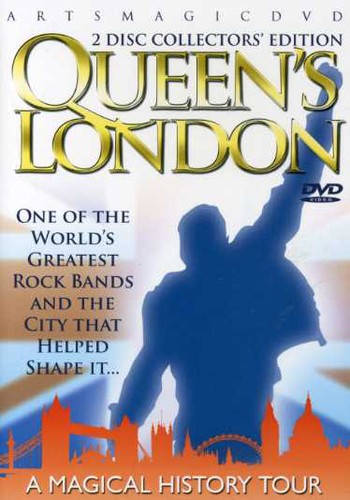This image is the cover of a two-disc collector's edition DVD titled "Queen's London," produced by Arts Magic DVD. At the top, against a white background, it reads "Arts Magic DVD" in black capital letters, followed by "Two Disc Collector's Edition" in smaller black capitals just above the word "Queen's." The main title, "QUEEN'S LONDON," is prominently displayed in large golden letters with black shadowing. Below the title, there's a DVD logo.

The cover features a blue silhouette of a person, likely a rock star, raising their right fist triumphantly. The figure, which lacks detailed features, appears to be on stage with their left arm hanging down and slightly out to the side, possibly wearing a jacket that flares out as the arm is raised. The silhouette is positioned primarily on the right side but extends across to the left.

To the left of the figure, the text reads in capital letters: "ONE OF THE WORLD'S GREATEST ROCK BANDS AND THE CITY THAT HELPED SHAPE IT." This text spans from the level of the figure's head down to its left elbow. In the background, a faint image of the British flag, the Union Jack, can be seen, adding a subtle touch of red, white, and blue to the design.

At the bottom of the cover, an orange outline depicts the London city skyline. The very bottom text reads "A MAGICAL HISTORY TOUR" in all capital white letters. The overall style of the cover combines elements of photography and illustration, creating a dynamic visual representation of both the band Queen and the city of London.